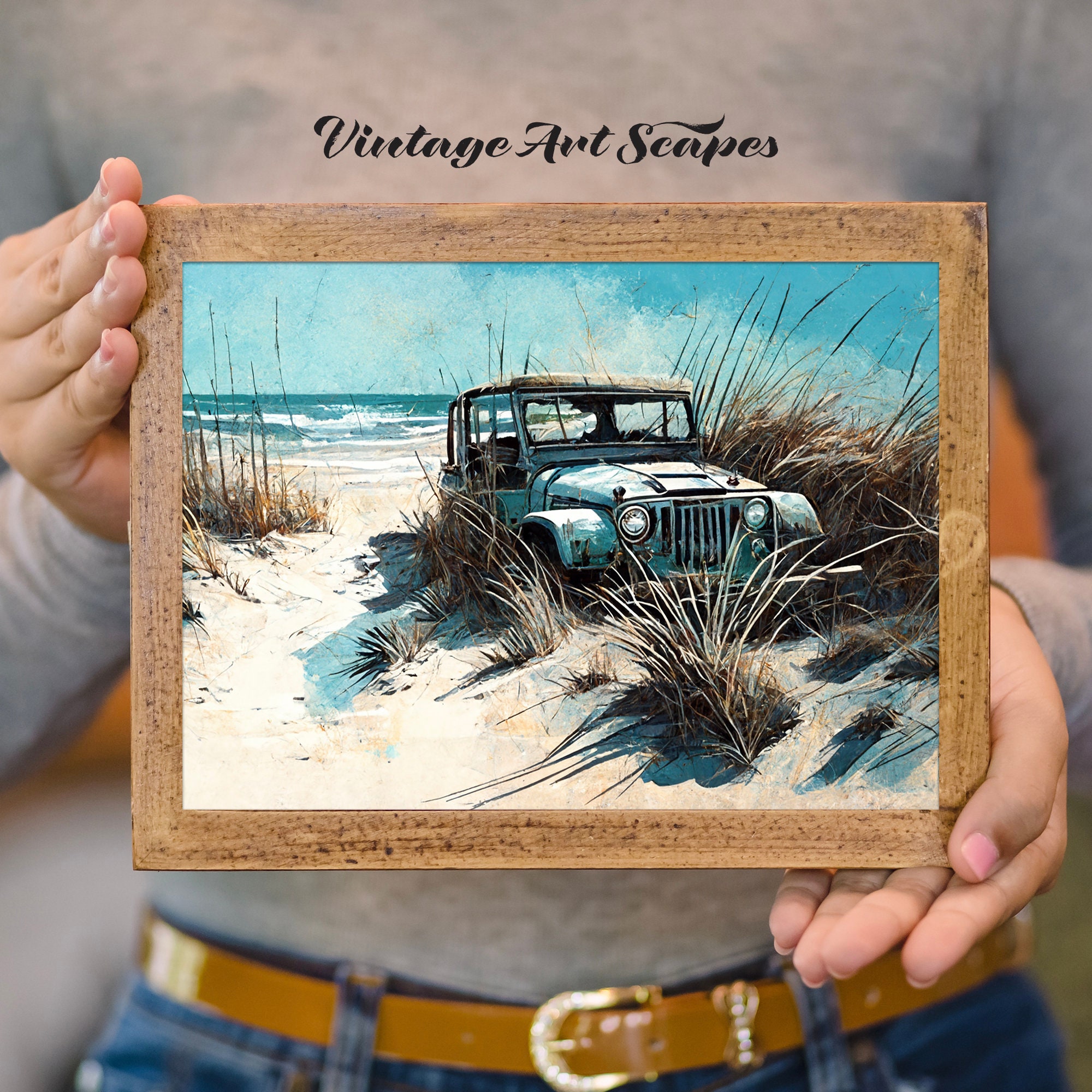In this detailed image, a woman with pink-painted eyebrows is holding a framed photograph. The frame is brown, and the woman's attire includes a long sleeve gray top, a brown belt with a gold buckle, and blue jeans. The text "Vintage Art Escapes" appears in black at the top, indicating an advertising piece or purchasable art. The photograph within the frame depicts a serene sandy beach scene, featuring light beige sand accented with sea grass and reeds. 

In the foreground, an older model Jeep, grayish and potentially rusty, sits parked among the grasses. The Jeep's headlights are white, and although it appears stationary, it is unclear if it's broken down. The background shows a dynamic ocean with active, rolling waves against a light blue or teal sky, adorned with whitish bits, possibly foam or reflections of light in the water.